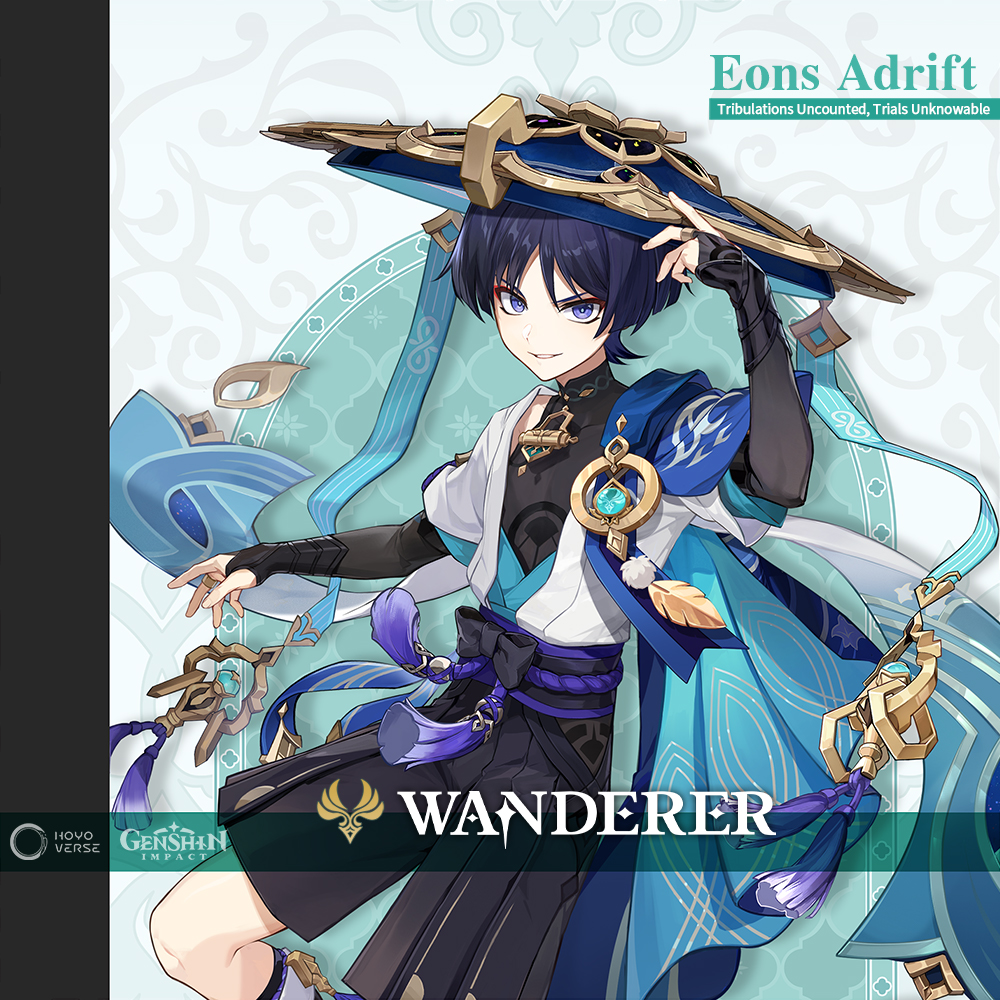The image features an anime-style illustration of a young boy, likely intended for a comic or video game. The artwork aligns with traditional Japanese anime aesthetics, characterized by oversized eyes and a narrow face. The boy is adorned with a distinctive hat reminiscent of a Vietnamese conical hat, featuring a wide brim and an ornate metallic design around its edge. The hat boasts a decorative, gold-colored flower at its peak.

The boy's medium-length black hair extends slightly past his ears. He is dressed in a black garment resembling a kilt, secured with a blue rope that forms a black bow at the front. Layered over a long-sleeve black shirt, he wears a white gi with a blue shoulder pad on his left side. The boy stands in a dynamic pose, facing the viewer, with his left hand adjusting his hat while his right knee is raised. The word "Wanderer" is displayed below him, perhaps signifying his character or role.